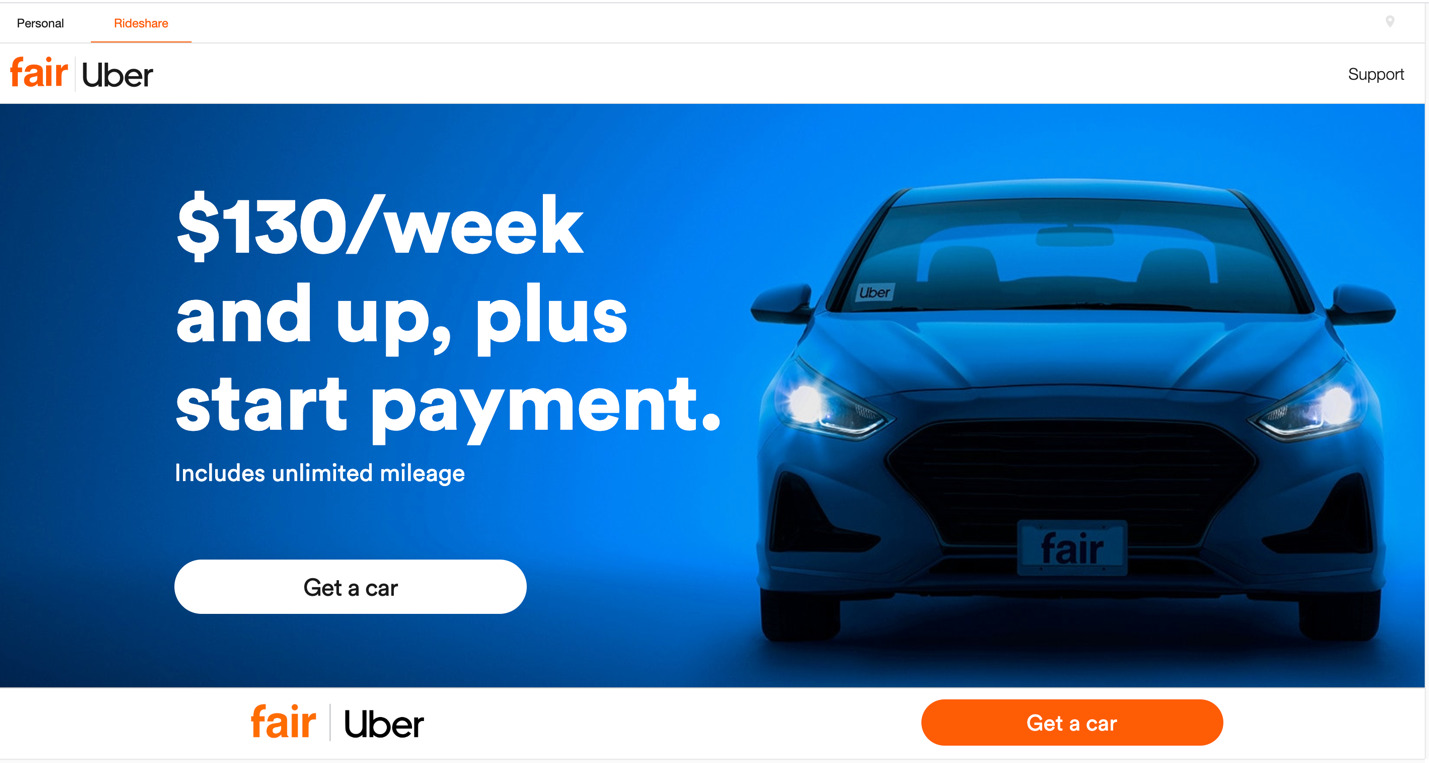At the top of the webpage, the word "Personal" is written in black letters. Adjacent to it, the word "RDShare" appears in red. Below this, there is a line of text featuring a red word followed by a black word, separated by a vertical gray line. The red word is "fare," and the black word is "Uber."

The main section of the page features a rectangle with a gradient background that transitions from bright blue to light blue to dark blue, moving from left to right. On the left side of this rectangle, bold white letters display a pricing detail: "$130/week, plus start payment." Below this, in smaller white text, it states: "includes unlimited mileage."

Also within this rectangle, there is a white, rounded rectangle with the text "Get a Car" written in black ink. Positioned on the right side of the rectangle is an image of a blue car, matching the blue shades of the background. The car appears to be a four-door sedan, with its headlights on and an Uber sticker located at the bottom left corner of the passenger side windshield. The car's license plate reads "fare."

Beneath this blue rectangle, on the right, there is a red, rounded rectangle that also says "Get a Car" in white letters. To the left of this, "fare" and "Uber" are written in the same configuration as above, with "fare" in red and "Uber" in black, separated by the vertical gray line.